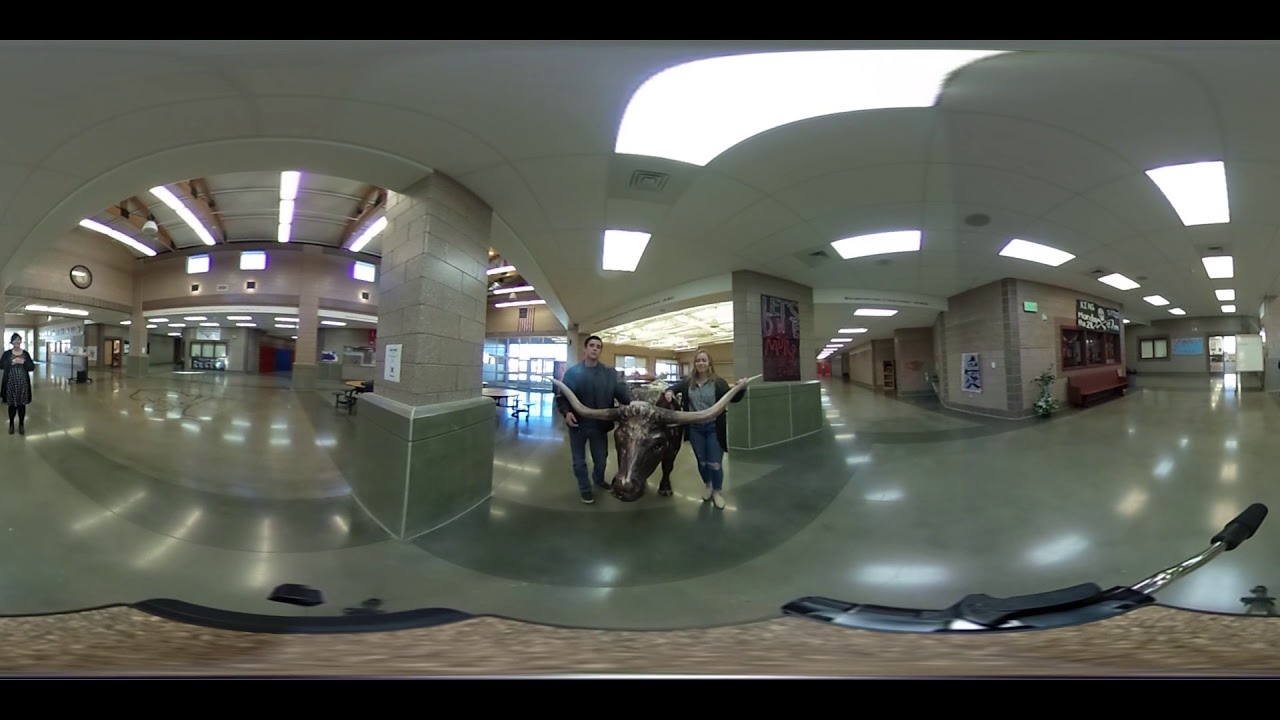In the center of this panoramic indoor image, there's a large bronze ceramic bull with long white horns, being held by a man and a woman. The man, standing to the left of the bull, is dressed in blue jeans and a blue shirt, while the woman to the right has long blonde hair and is wearing jeans with tears in the knees, along with a green overshirt over a gray undershirt. The floor beneath them is an alternating pattern of dark and light gray, reflecting the numerous overhead lights. The area is spacious, likely an atrium or museum with a high, white ceiling. 

To the far left, another woman in a black skirt is walking towards the camera. Just behind her, there's a tile or brick post. On the right side of the image, a booth with a black banner featuring a white Jolly Roger and partially legible word "king" is visible. Nearby, a red bench is positioned against a tan or gray wall, and various posters are displayed. Amongst this, sticks resembling handlebars or selfie sticks can be spotted, suggesting the photo might have been taken from a bike or similar device. The building's interior features a mix of gray and tan tones, and there are hints of red and blue areas further in the background. The outdoor light streams in from the left and mid-right sections of the building, enhancing the indoor ambiance.